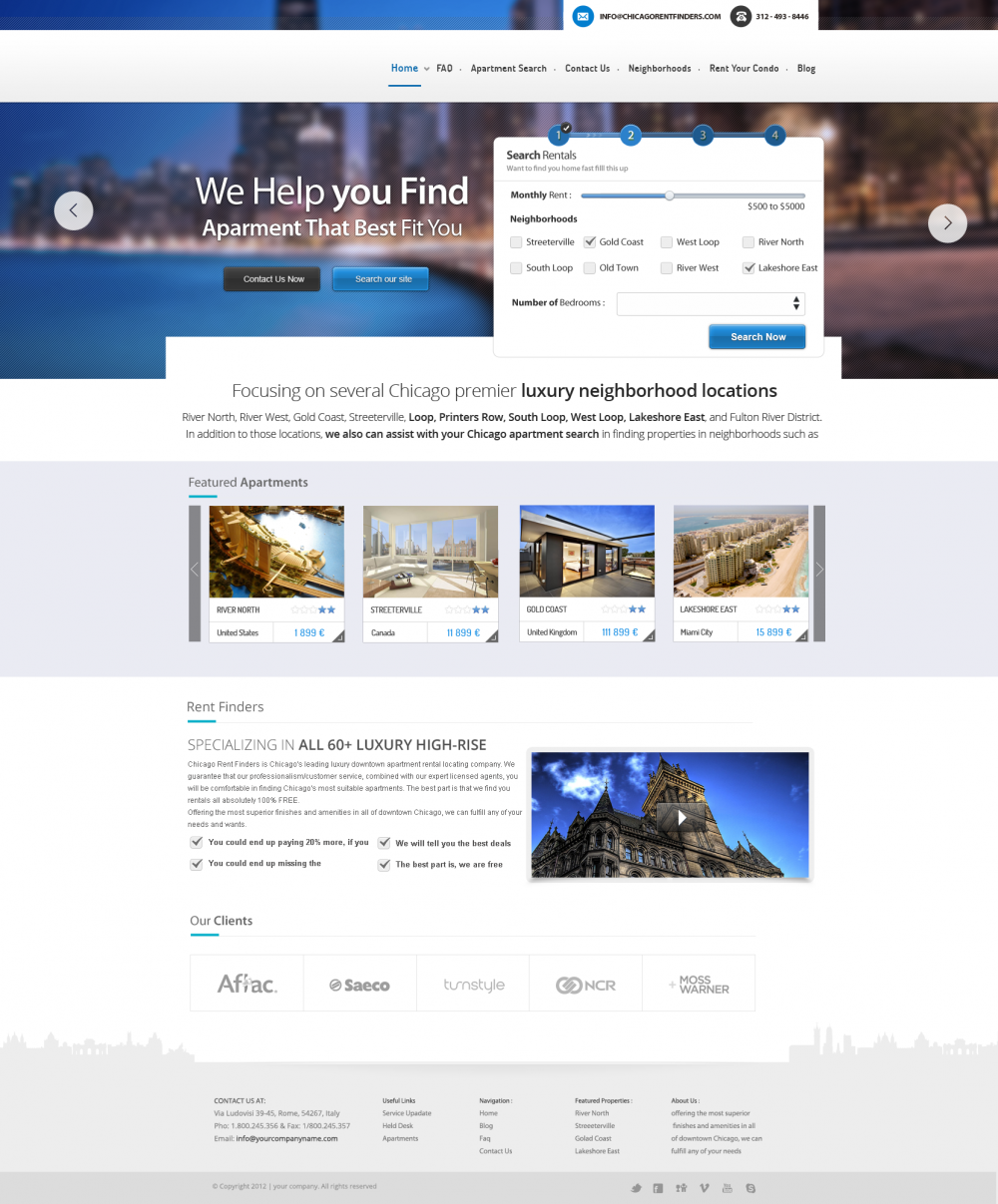This web page is designed for apartment seekers, showcasing various rental options across different neighborhoods. At the top of the home page, there's a rotating photograph banner that users can click to view multiple images. Directly above this banner, users can access the main navigation tabs: Home, FAQ, Apartment Search, Contact Us, Neighbors, Rent Your Condo, and Blog. 

To the top right, there’s a circular icon with a white phone image on a black background, accompanied by a phone number for easy contact. The search functionality allows users to filter apartments by streets or various regions.

As you scroll down, the page highlights apartment listings with detailed photos and descriptions. Currently, it showcases luxury neighborhood locations with options listed numerically (1, 2, 3, 4). Each listing includes a high-quality image of the apartment or building, its neighborhood (such as Gold Coast, Streeterville, or River North), the country, and the rental price. 

Below these listings, there’s an example segment explaining Rent Finder's specialty in over 60 luxury high-rise apartments, providing more detailed information about their services.